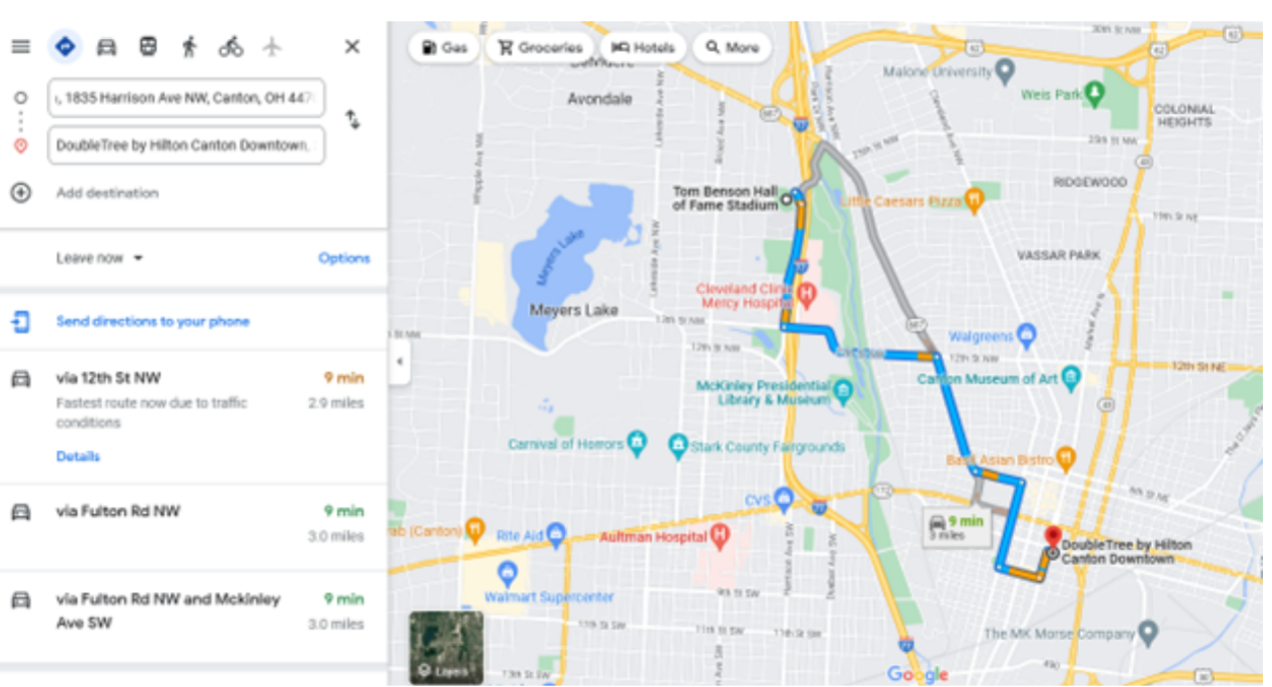A search results page from Google Maps displays directions from 1835 Harrison Avenue Northwest, Canton, Ohio. On the right side of the screen, there is a detailed map, while the left side lists various route options. The top search bar prominently shows the address searched. One of the highlighted destinations is DoubleTree by Hilton Canton Downtown. Below, options for navigation appear, with selections like "Leave Now" and the ability to send directions to your phone. 

The fastest route suggested takes approximately nine minutes via 12th Street Northwest, covering 2.9 miles. Alternative routes include Fulton Road Northwest, also nine minutes but 3.0 miles, and a combined route via Fulton Road Northwest and McKinley Avenue Southwest, each taking around nine minutes. The directions are displayed with colored route lines - blue, red, yellow, orange - and the map background includes shades of green, gray, black, and white. In the bottom-left corner is a small, thumbnail photo map overlaying the main drawn map.